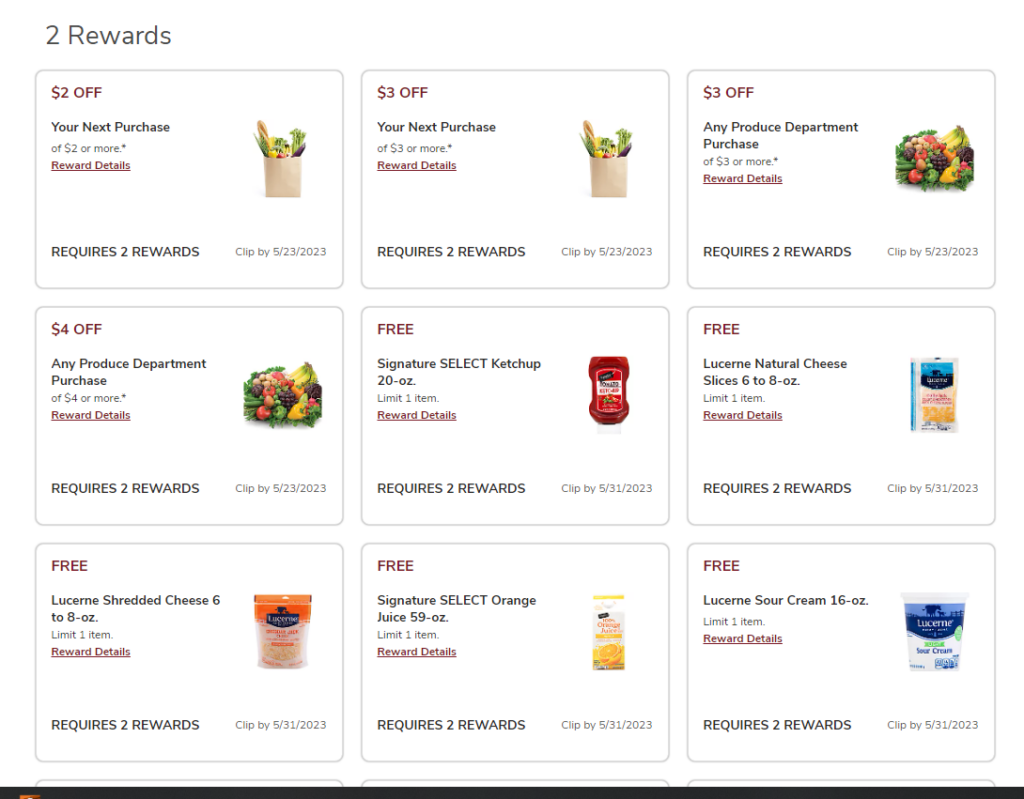This is a detailed caption for an image that appears to be a screenshot from a grocery store rewards app. The background is white, and at the top, in black font, it reads "Two Rewards" situated on the upper left. Below this heading are three rows of three selections, each bordered by a black line, forming squares.

In the first row:
1. The first selection on the upper left offers "$2 off your next purchase of two or more" and requires two rewards. Accompanying this text is a small photo of a shopping bag.
2. To the right, the second selection displays "$3 off your next purchase of three or more" and also requires two rewards. This too features the same shopping bag image.
3. The final selection on the upper right offers "$3 off any produce department purchase" and requires two rewards. It includes a photo of a table of fruit.

In the second row:
1. The first selection on the left offers "$4 off any produce department purchase of four or more" and requires two rewards, using the same fruit table image as before.
2. To the right, the second selection features "Free Signature Select Ketchup 20 ounces," which requires two rewards. There's a picture of a ketchup bottle alongside this offer.
3. The final selection on the right provides "Free Lucerne Natural Cheese Slices 6 to 8 ounces," requiring two rewards. Next to the description is a picture of a package of cheese slices.